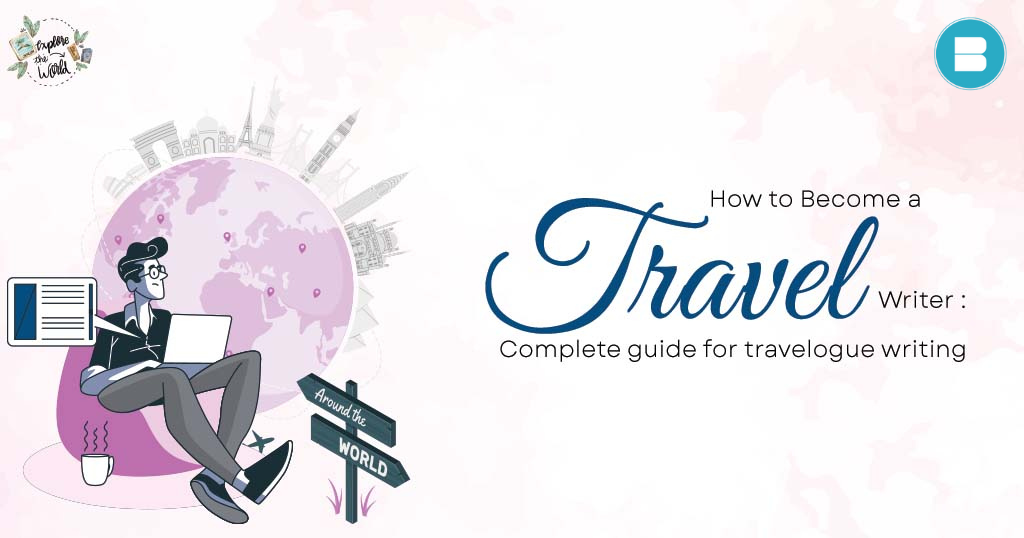The illustration for the "Around the World" ad features a detailed and vibrant design set against a swirling pink watercolor background. A grayscale man wearing glasses is depicted typing on a laptop, comfortably seated on a pink beanbag with a mug of coffee beside him. The focal point, immediately behind the man, is a pink watercolor-style Earth showcasing iconic world landmarks in grayscale, including the Eiffel Tower, Tower of London, Statue of Liberty, and the Colosseum, among others. Beside him are wooden signs embedded in the ground that read "Around the World". The top left corner displays a logo with the same phrase. The main text on the white background states, "How to Become a Travel Writer: Complete Guide for the Travelog Writer," and there's a subtle detail of an airplane taking off near the man's left leg. Additionally, a watermark in one corner of the image reads, "Explore this world."